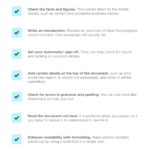The image features a series of seven light blue squares, each positioned along the right and left sides of the composition. Inside each square is a dark blue check mark. The central part of the image contains text displaying the names of various senses, though it is slightly blurry and written in small, black font, making it somewhat difficult to read. The entire illustration is set against a clean, white background.